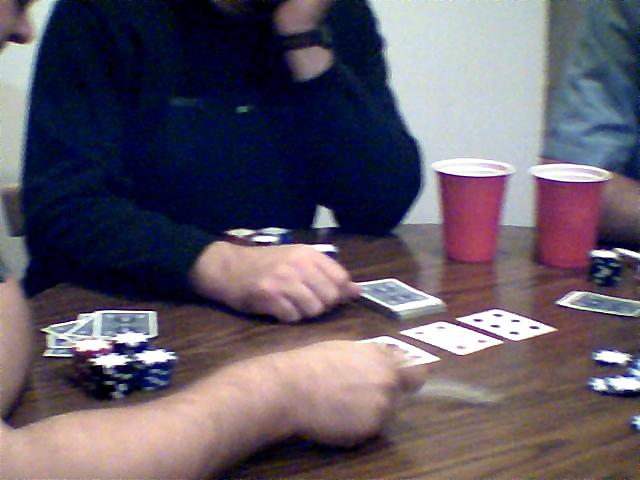The image portrays a casual, intimate scene of three individuals engaged in a card game around a circular table. The photograph, slightly grainy and pixelated, seems to have undergone digital enhancement, lending an unnatural hue to the shirt of the man in the background. The table is cluttered with red solo cups and neat piles of poker chips, indicating an ongoing game. Spread out on the table are a six of spades, a four of diamonds, and a face-down court card, hidden under the hand of one of the players. The person on the left, only partially visible from the arm and elbow, appears to be in the midst of placing a card down. The background player, donning a peculiarly tinted blue shirt, has a contemplative posture with his fist resting on the table, likely supporting his chin with his left hand. The player on the right rests his right arm on the table, though much of it is obscured by one of the solo cups. The scene, albeit captured in lower quality, vividly depicts the relaxed, concentrated atmosphere of a friendly card game.